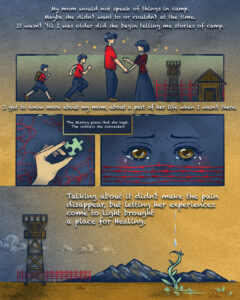The image appears to be an illustrated page from a children's storybook, divided into three distinct sections. The overall color palette is dominated by gray and yellow hues, reminiscent of a yellow-orange sky with gray clouds sprinkled with stars. The top section features white text against the sky, slightly blurred and difficult to read, but it conveys a poignant message: "My mom would not speak of things in camp; maybe she didn't want to or couldn't at that time. It wasn’t until I was older that she began telling me stories of camp."

Below this, the middle section is divided into two parts. On the left, two young children are running, while on the right, two teenagers, a boy, and a girl, are holding hands, gazing at each other from a side profile. Flanked to their right are nondescript buildings. This section subtly transitions into the lower part of the page.

At the bottom, the illustration shifts to a landscape featuring a large tower with a cabin on top, positioned to the left, and mountains to the right. The foreground showcases brown soil from which a plant is growing, with water droplets visible. Text overlays this scene, stating, “It didn't make the pain disappear, but letting her experience come to light brought a peace place for healing.”

Additionally, within the image's middle section are two contrasting insets: one on the left shows a hand holding a blue jigsaw puzzle piece against a black background with red threads or ribbons, while the other on the right depicts a crying face with yellow eyes and red lines beneath them. These segments are connected by a text box that is too blurred to decipher.

Together, the vivid illustrations and heartfelt text narrate a story of personal history, emotional healing, and the journey towards understanding and overcoming past traumas.